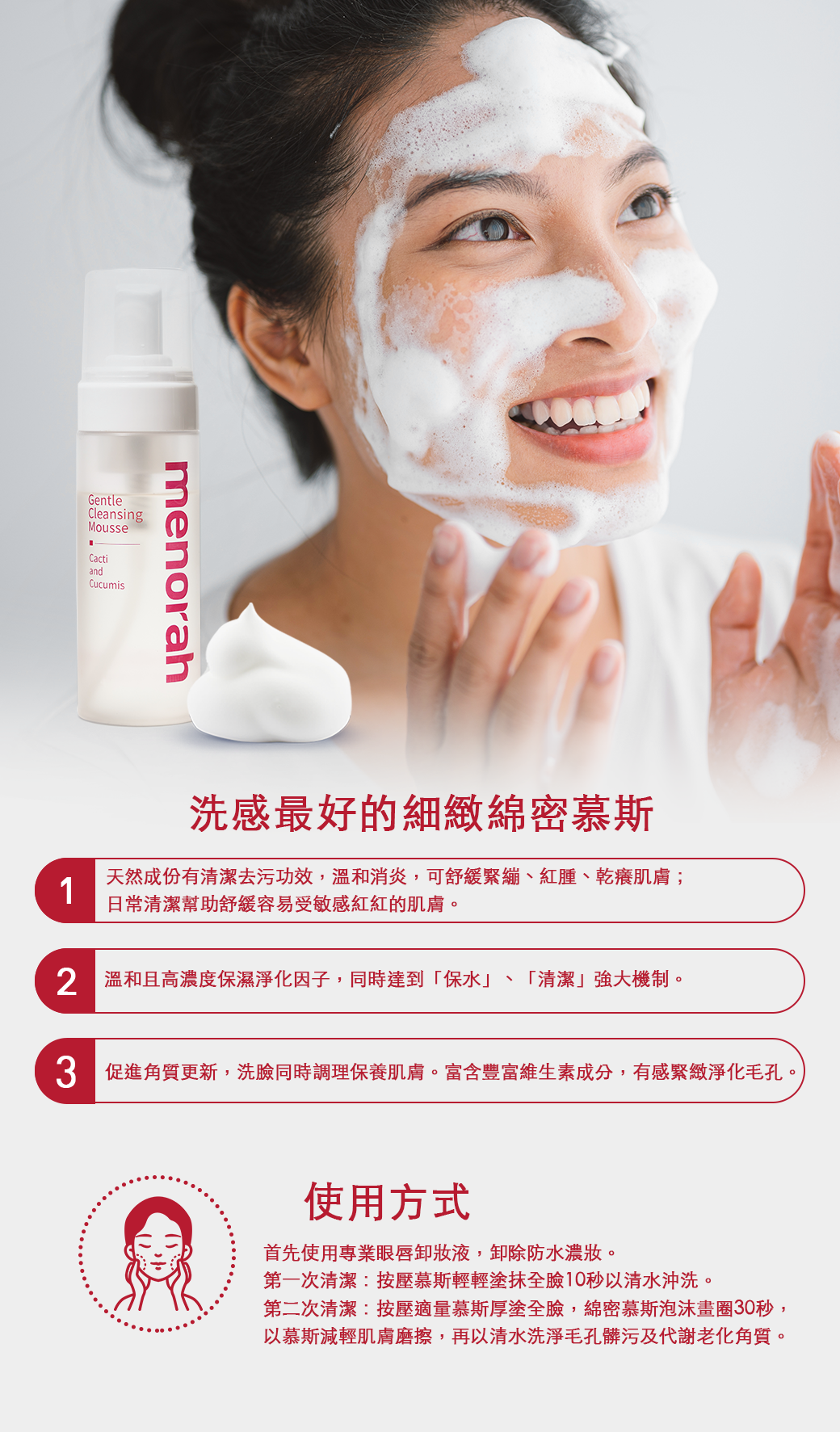The photograph depicts an advertisement for Menorah, a gentle cleansing mousse. The focal point is a Chinese-descended woman with dark hair tied up in a bun, showcasing the product on her face with a happy expression. The white cylindrical bottle of the mousse, featuring a reddish pink "MENORAH" label and a pump, is positioned on the left side. The bottle sits next to a pile of foam resembling shaving cream. The woman has applied the mousse across her forehead, cheeks, nose, and chin. Surrounding the main image, there are detailed instructions in Chinese characters, highlighted in a red color matching the bottle's label. The instructions are segmented into three bulleted areas, numbered one, two, and three, providing further details on the product’s usage.